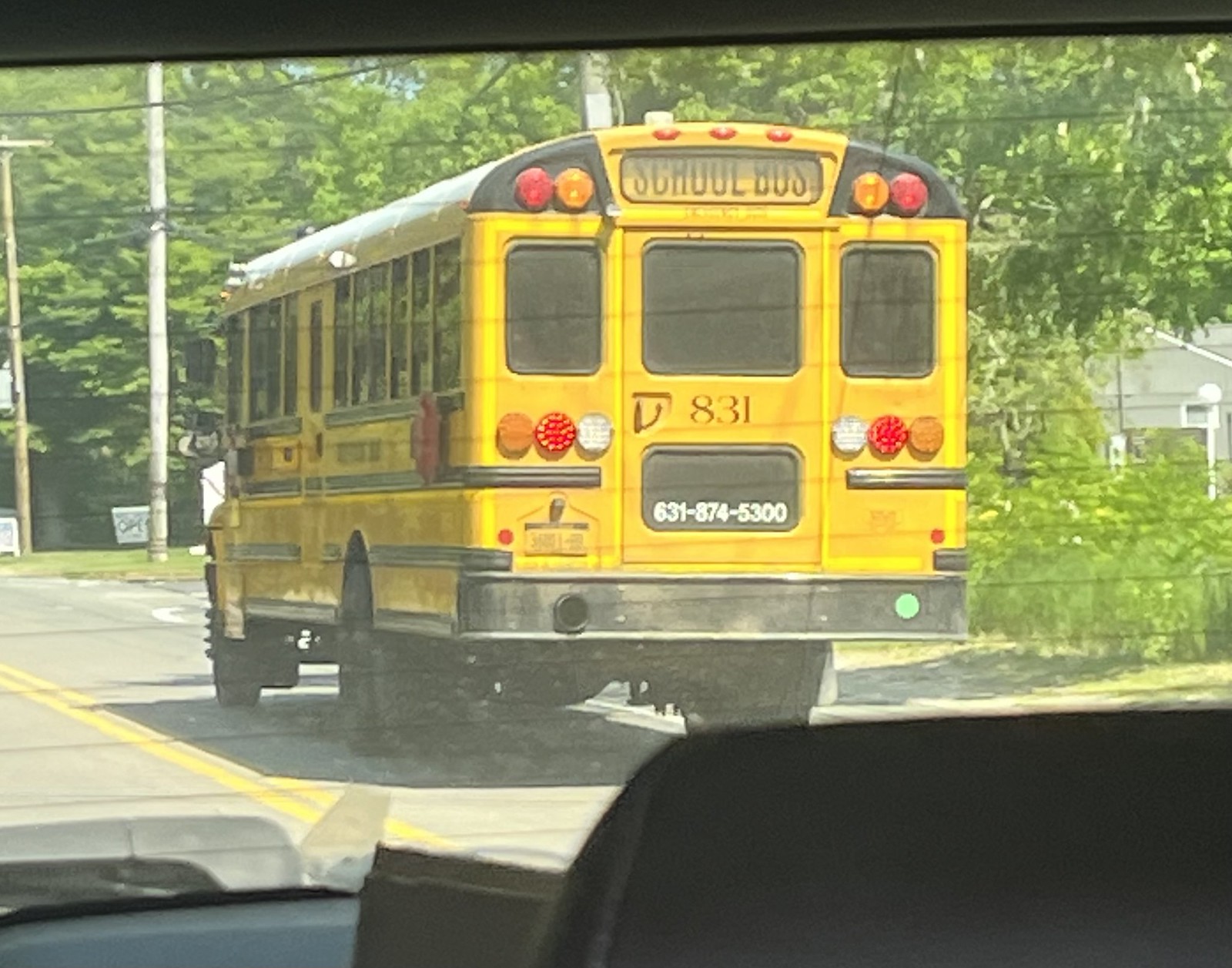This detailed photograph captures the rear end of a large yellow school bus numbered 831, taken through the back window of another vehicle with defrosting strips visible across the rear windshield. The bus, adorned with multiple colored lights including red, orange, and white, is situated on a gray road marked with yellow striping and white lines, indicative of a residential neighborhood. Surrounding the scene are green trees, shrubbery, and a light gray house to the right. The bus's sign above the back door reads "School Bus," and a phone number displayed on the bottom window says "631-874-5300." Additionally, there's a yellow license plate with a blue stripe on the bottom left, reminiscent of New York plates. On the passenger side of the bus, a stop sign is visible, utilized when loading or unloading children. The scene is likely set during the daytime, with the bus positioned towards the left side of the photograph, driving or possibly stationary, on a road flanked by telephone poles. A black seat is also faintly visible in the bottom right corner of the image, indicating the photo was taken from inside another vehicle.